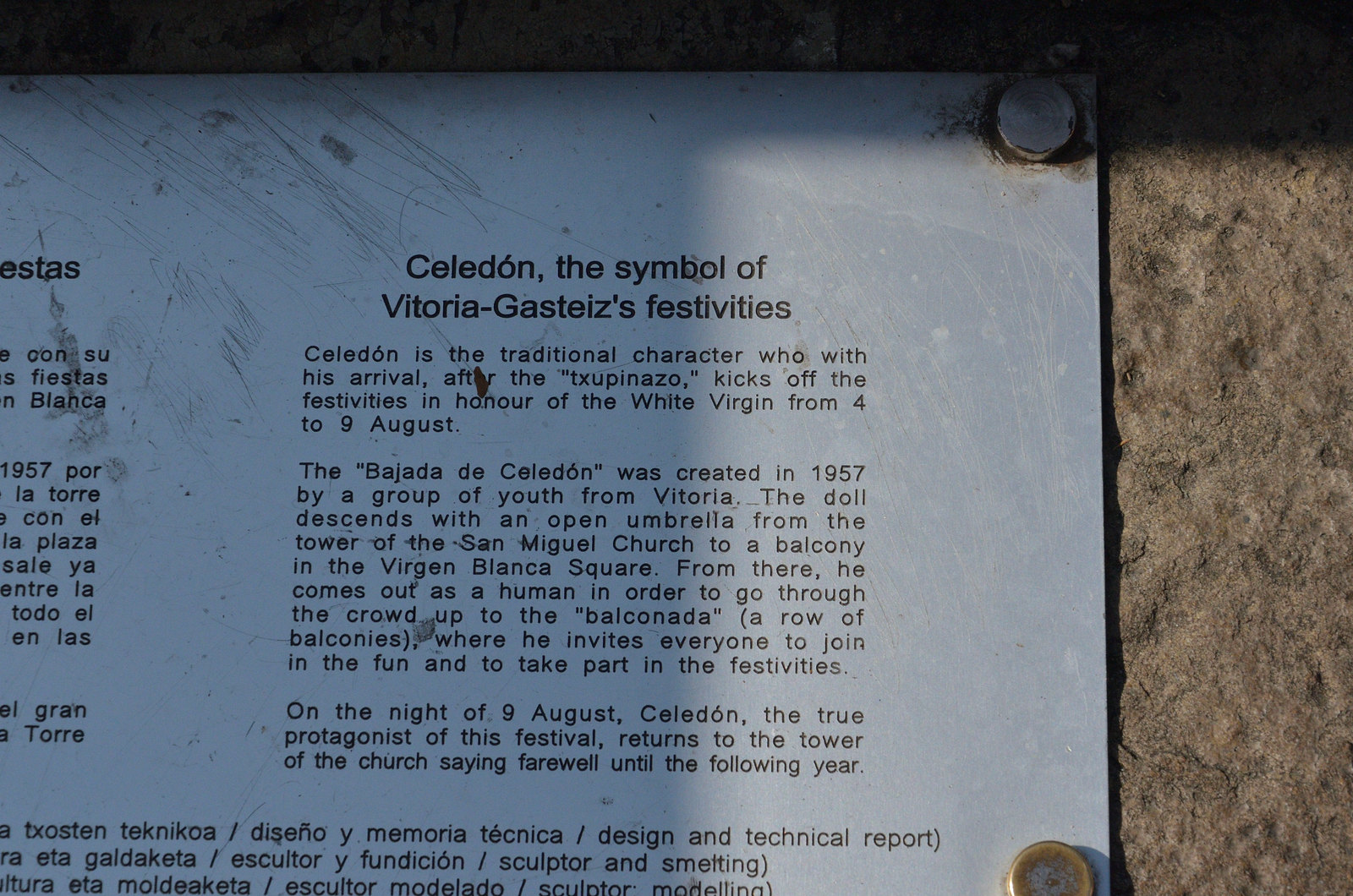This close-up color photograph captures the corner section of an informational plaque bolted to a gray stone surface. The plaque is made of plain silver steel metal with black text. It describes "Célédon," the symbol of Vitoria-Gasteiz's festivities. Célédon is a traditional character whose arrival after the "txupinazo" (basque for rocket or fireworks launch) inaugurates the festivities in honor of the White Virgin, taking place from August 4th to 9th. Created in 1957 by a group of local youth, the plaque narrates how a doll of Célédon descends with an open umbrella from the tower of the San Miguel Church to a balcony in the Virgen Blanca Square. Upon landing, Célédon transforms into a human form, weaving through the crowd up to the "balconata," a row of balconies, where he invites everyone to join in the celebrations. On the night of August 9th, Célédon, the main protagonist, returns to the church tower, marking the end of the festivities until the following year. The photograph shows only part of the plaque, with some additional text being cut off.